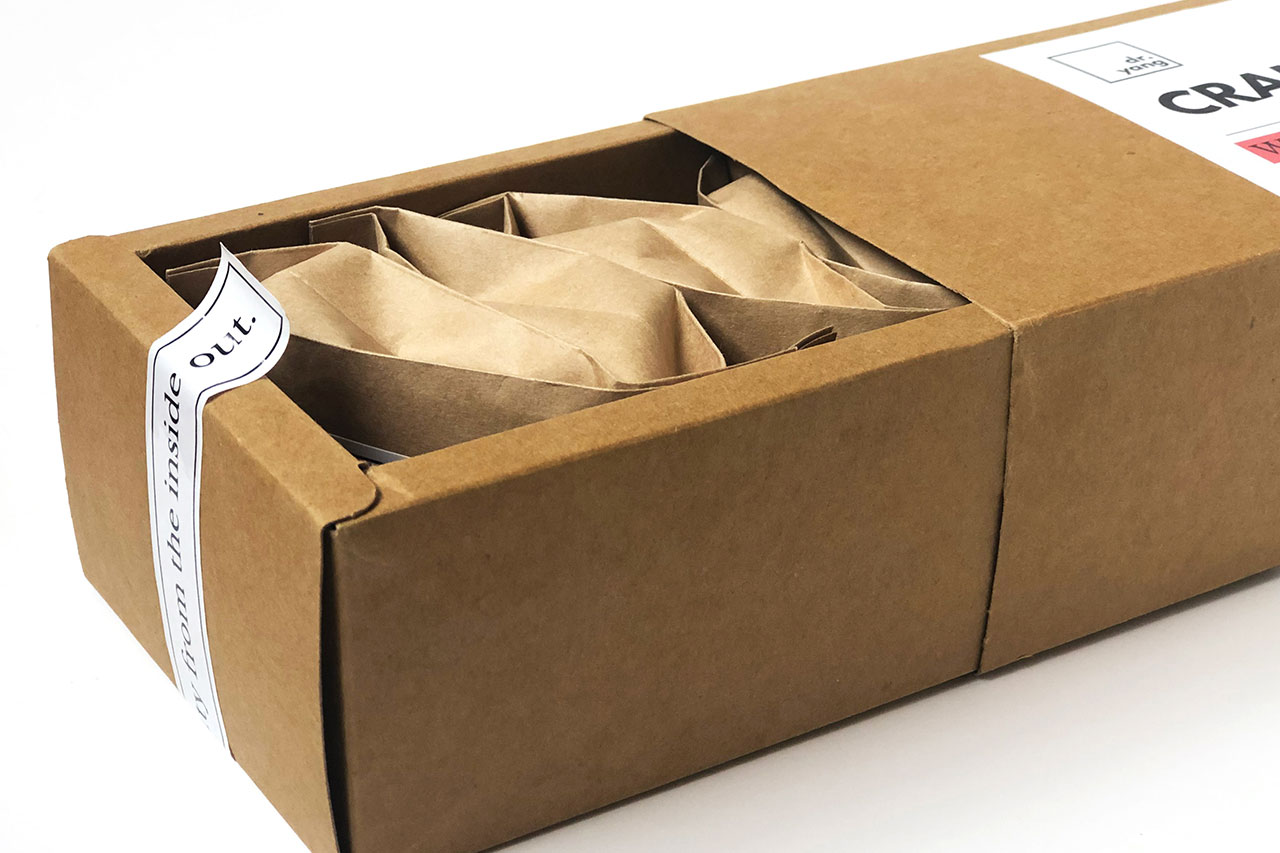The image depicts a rectangular cardboard box approximately six inches wide and four inches high, set against an off-white background. The box, with an open top, is partially pulled out from its slipcover, which moves from the upper right corner diagonally towards the lower left. Inside the box are small packages, each wrapped in light brown paper. A prominent white label is affixed to the box's top right hand corner, containing the text "Dr. Yang" in a small square, with the bold black letters "CRA" beneath it. Additionally, a white sticker on the box's exterior reads "from the inside out." The overall composition draws attention to the detailed packaging and labels.